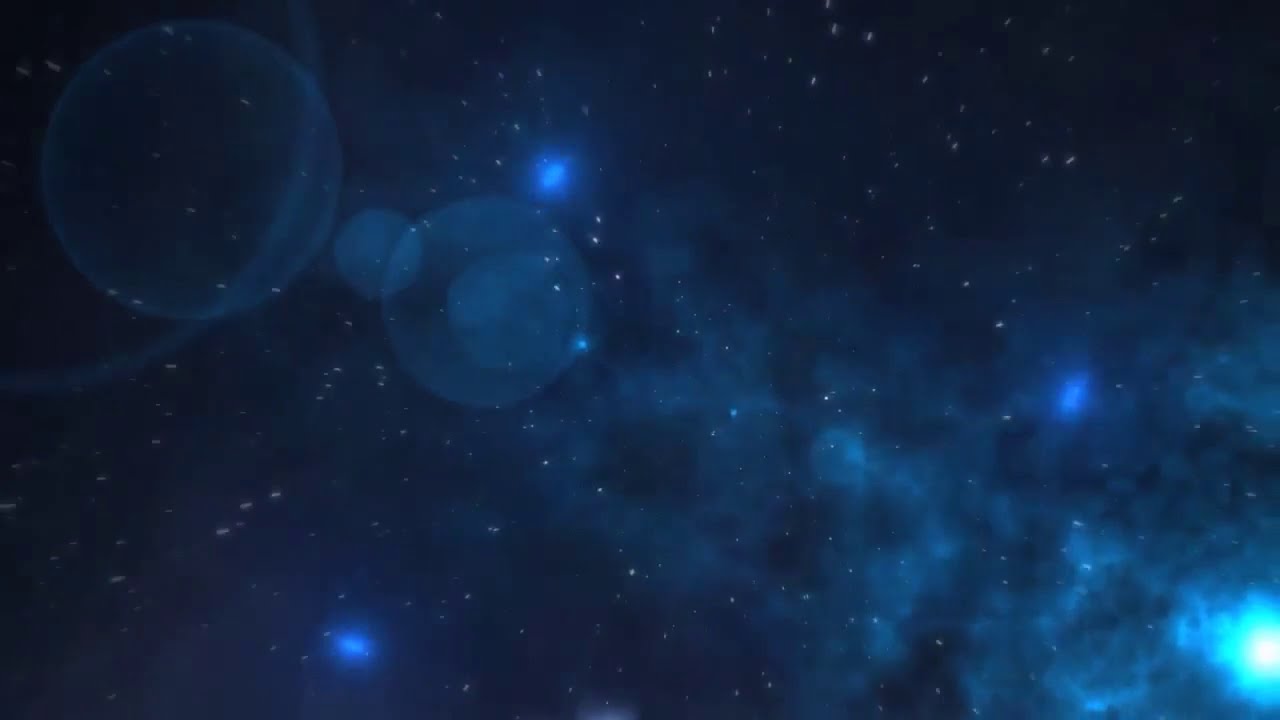The image presents a digitally-created representation of the night sky, evoking a sense of cosmic wonder. The backdrop is a gradient of deep navy blue to black, studded with numerous stars of varying sizes and brightness, mimicking the natural night sky. Intermittent thin clouds traverse the scene, adding to its ethereal feel. In the bottom right corner, there's a prominent bright blue light with a white core, accompanied by a misty trail, suggesting motion. This feature, along with other scattered blue highlights forming a subtle triangular pattern, enhances the image's celestial depth. The top left corner also contains several reflective circle-like dots, reminiscent of viewing through a telescope. These elements collectively create an intricate and detailed depiction of outer space, blending artistic creativity with astrological aesthetics.